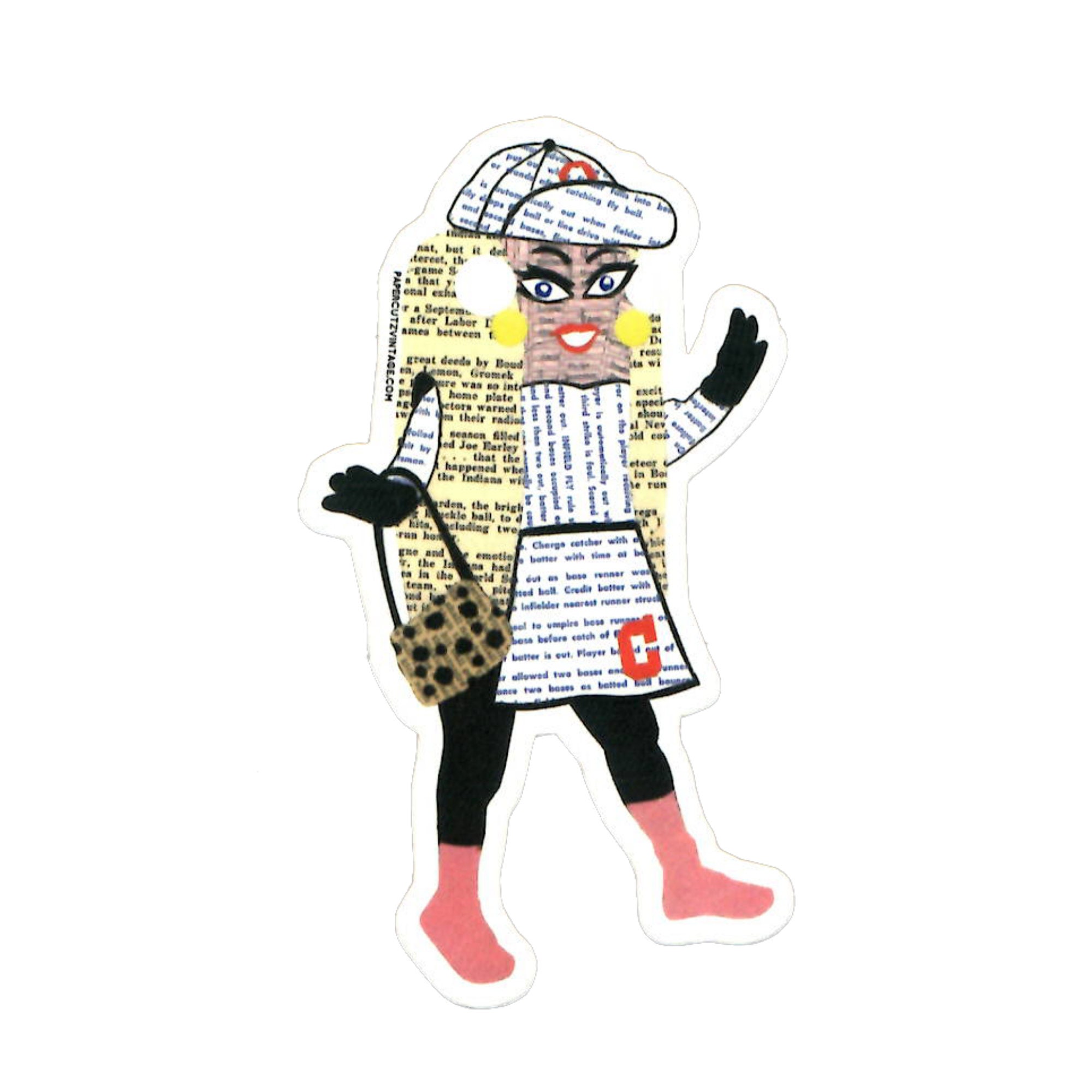The image is a detailed collage of a woman, meticulously crafted from cut-out snippets of newspaper or book pages with small text. The woman is accessorized with prominent yellow earrings and wears a unique baseball hat with its brim turned upwards, possibly adorned with a red capital letter C. Her face, composed of various paper fragments, features rectangular proportions, dark blue eyes accentuated with heavy mascara, and striking red lips. She sports cat-eye glasses, adding to her quirky appearance. 

The woman is dressed in a distinct yellow jacket, paired with a white skirt that features a prominent red capital C. She holds her arms out to her sides, with a leopard print purse hanging from her right wrist. Below, she is clad in black leggings and dons pink socks or boots on her feet. Additionally, there's an unexplained large white dot to the left of her eyes. The entire figure embodies a playful yet sporty aesthetic, resembling a woman preparing for a game while reveling in a shopping spree, all painstakingly brought to life through a collage of text-laden paper pieces.